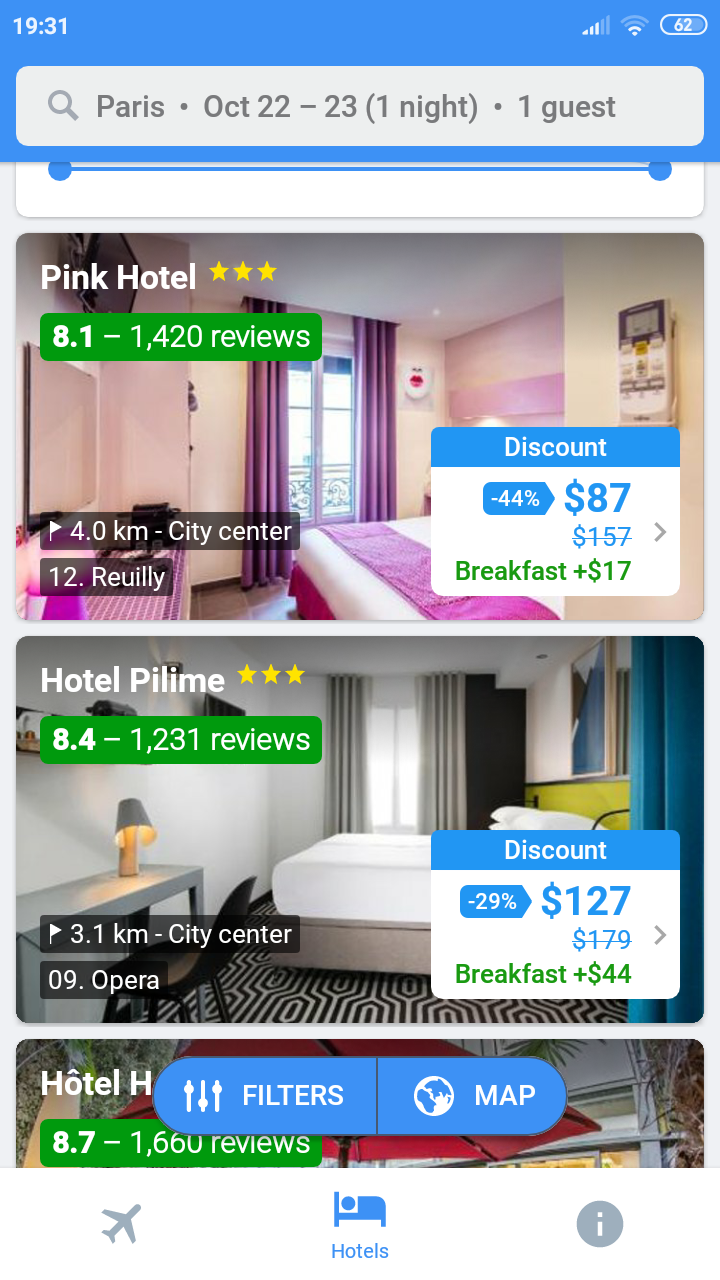A smartphone screenshot displaying hotel discounts is depicted, featuring a blue upper border with a timestamp of 19:31 in the top left corner. Complementing the interface, the top right corner shows a Wi-Fi icon and a battery indicator at 62%. Immediately below lies a search box labeled "Paris, October 22nd through 23rd (one night • one guest)."

The first hotel listed showcases an image of a mid-grade room in the Pink Hotel, boasting a three-star rating with an 8.1 score from 1,420 reviews. A flag icon denotes its distance from the city center as 4.0 kilometers. Prominently, a discount label indicates a significant price drop from $157 to $87, offering a 44% savings, with an optional breakfast available for an additional $17.

Next, Hotel Pilemi, a similarly mid-grade establishment, is presented with a three-star rating and an 8.4 score from 1,231 reviews. The flag icon here highlights a 3.1-kilometer distance from the city center, specifically zero nine opera. A discount tag reveals a reduction from $179 to $127, marking a 29% savings, with breakfast priced at an extra $44.

Finally, an entry for another hotel (name partially obscured), rated 8.7 based on 1,660 reviews, is visible. Below these listings are tabs for filters and a map, accompanied by icons for flights, hotels (which is the current tab), and information in a silver circle at the bottom.